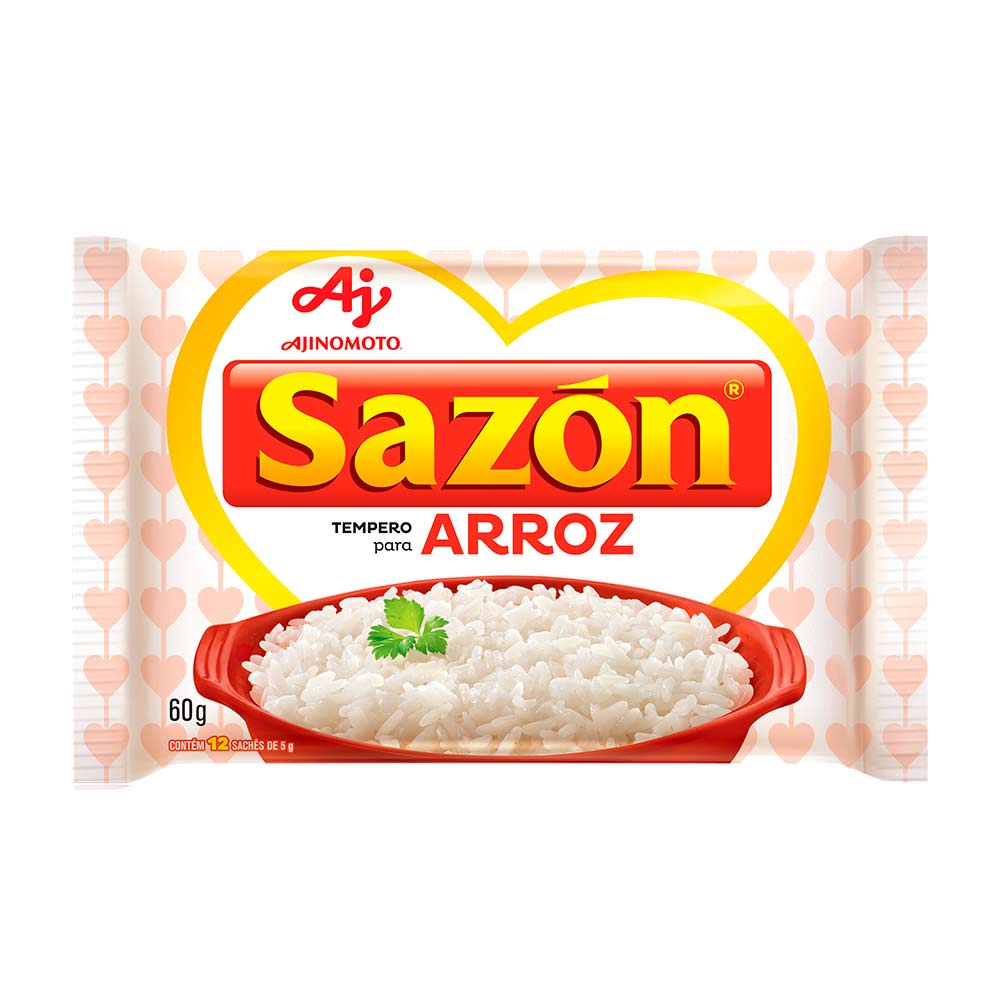The image depicts a bag of rice, primarily colored in white with scattered pink and red hearts, and a prominent yellow heart in the center. The rice, presented in a red bowl topped with a sprig of parsley, is positioned centrally on the package. Displayed on the heart-shaped label, the packaging text reads "Sazon Tempero para Arroz" by A.J. Ajinomoto and indicates a weight of 60 grams, which is said to make 12 servings. The photo also highlights the use of various colors including red, yellow, white, peach, green, and black, set in a product image style suitable for a food website.